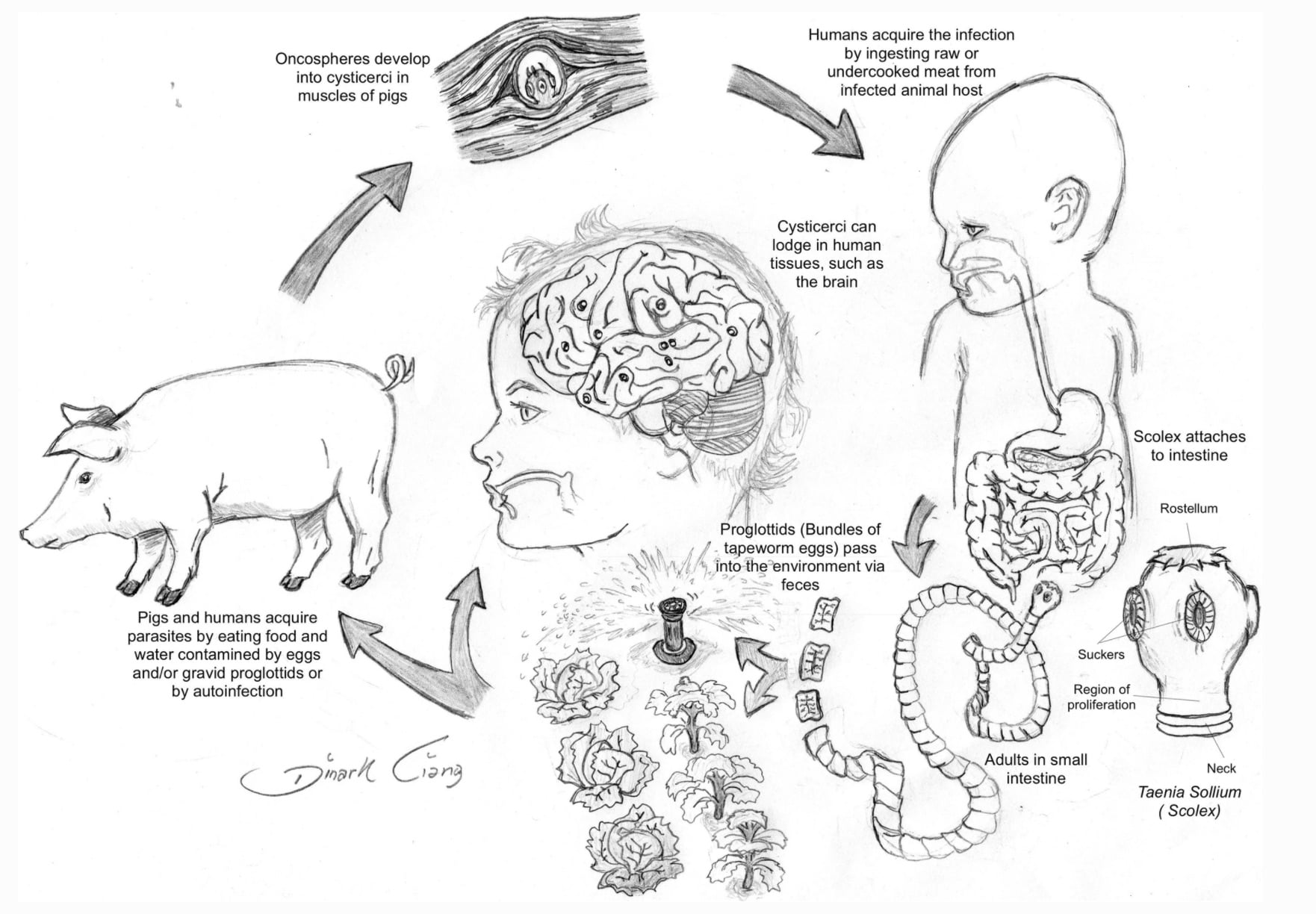The image depicts a detailed hand-drawn chart with a white background illustrating the transmission cycle of parasites between pigs and humans. On the left, there is a drawing of a pig, indicating that pigs and humans can acquire parasites by consuming food or water contaminated by parasite eggs or gravid proglottids, or through auto-infection. An arrow points from the pig to a depiction of parasite development in pig muscles. The chart transitions to the right where there is an image of a human, showcasing both the digestive and nervous systems. It highlights how humans ingest contaminated meat, leading to intestinal infection, and how the parasites can subsequently lodge in human tissues such as the brain. There are arrows and labels detailing each stage of the infection process, illustrating the progression from ingestion to the impact on human health. The central part of the image underlines the severe potential consequences, including brain involvement, depicted through spots in a drawn brain. This informative diagram clearly maps out the parasitic lifecycle, emphasizing the shared routes of infection between pigs and humans.